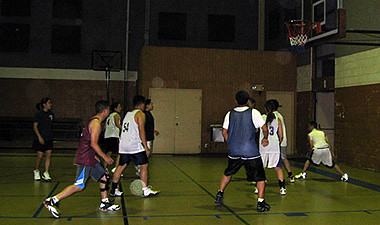The image depicts the interior of a brightly-lit gymnasium, clearly marked with basketball court lines and emblematic designs on the polished wooden floor. Several individuals are actively engaged in a game of basketball, forming what appears to be a co-ed team. The players, who seem to be of Caucasian descent, include both male and female participants. One female player is dressed entirely in black, adding a stark contrast to the scene. A male player is seen wearing a purplish jersey paired with bluish shorts, while another male player dons a white jersey with the number "34" emblazoned on the back, complemented by black shorts. The energetic atmosphere and dynamic movements of the players convey a sense of intensity and teamwork.